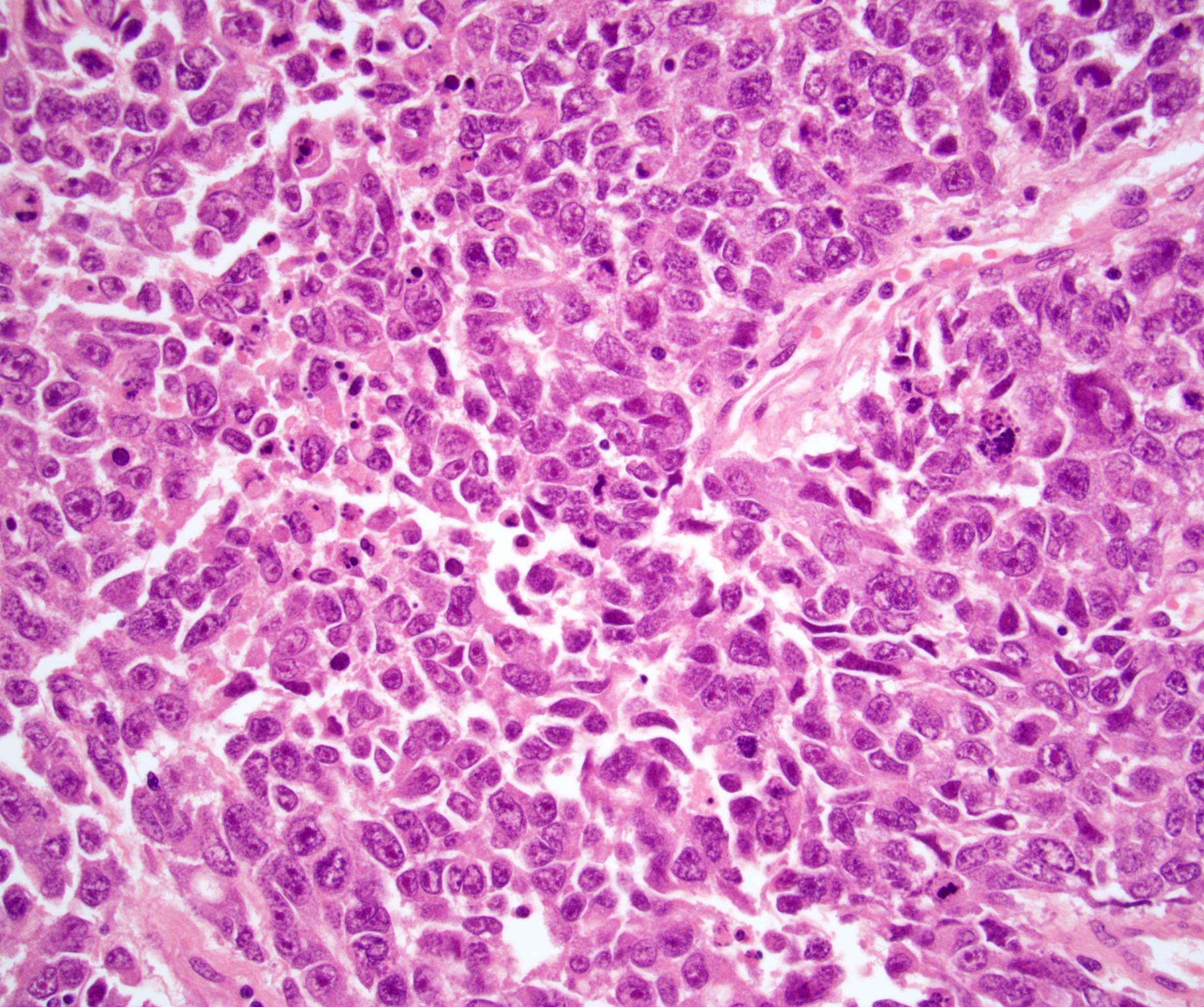The image is a detailed, pinkish-purple square that closely resembles a microscopic view of cellular structures, possibly blood or bacteria under a microscope. It is dominated by various rounded forms that mimic the appearance of cells or nodules, each uniform in color yet differing subtly in shade and shape—ranging from oblong to circular, and from clustered to isolated. Interspersed among these cellular shapes are delicate, light pink veins that run in multiple directions, akin to the veining seen in marble. The overall effect is a dense field of tiny purple cells with streaks of light pink, giving the impression of observing a sample teeming with life forms through a microscope.